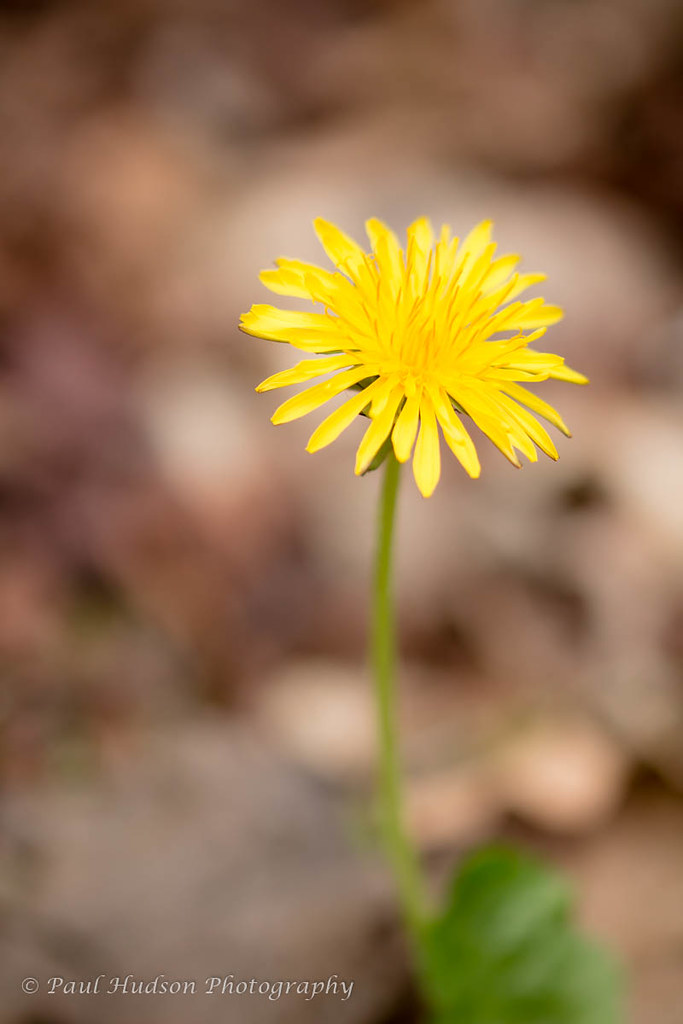The photograph features a vivid yellow flower with numerous petals, likely a dandelion or a daisy, perched on a green stem with a single leaf. The background is significantly blurred, revealing indistinct shapes that suggest rocks or a leafy ground, which enhances the focus on the vibrant flower. The portrait-oriented image, taller than it is wide, bears the watermark "Paul Hudson Photography" with a copyright symbol in the bottom left corner, solidifying its authenticity. The overall composition highlights the flower's intrinsic beauty against a soft, earthy backdrop.